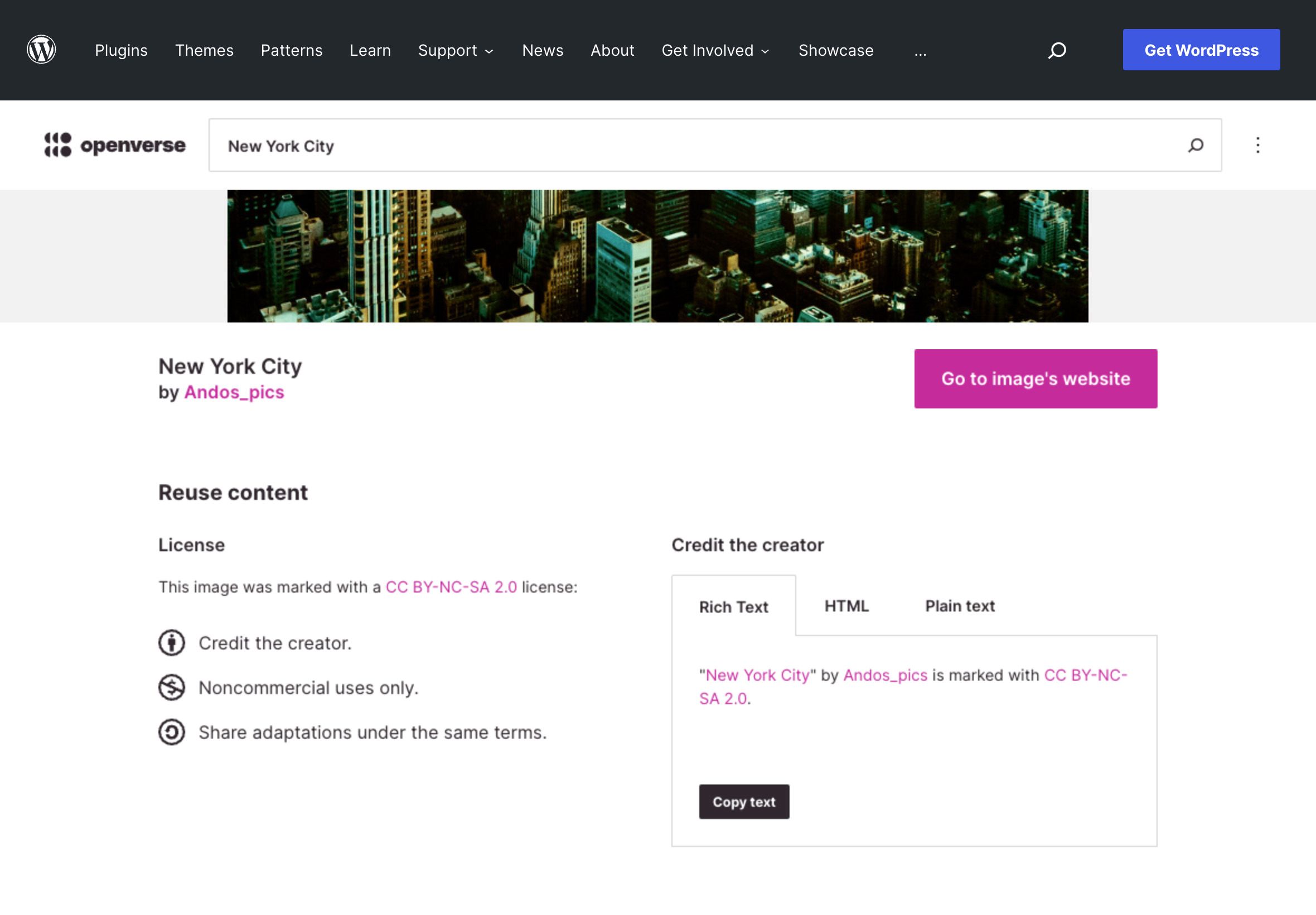In the screenshot, a dark gray navigation bar is displayed at the top, featuring several clickable options: Plugins, Themes, Patterns, Learn, Support, News, About, Get Involved, and Showcase. Additionally, there is an ellipsis ('...'), a search icon, and a prominent blue button labeled "Get WordPress."

Below this navigation bar, on the left side of the screen, there is a section labeled "Openverse" accompanied by a search bar with the placeholder text "New York City." Directly beneath this, a partial image is visible, depicting the top of buildings in New York City. The image is credited at the bottom left as "New York City" by the user Ando's_pics.

To the right of the image, a pink button labeled "Go to Image's Website" is prominently displayed. Furthermore, there is textual information regarding the image's license, stating, "Reuse Content. License: This image was marked with a CC BY-NC-SA 2.0 license. Credit the creator, non-commercial use only, and share adaptation under the same terms."